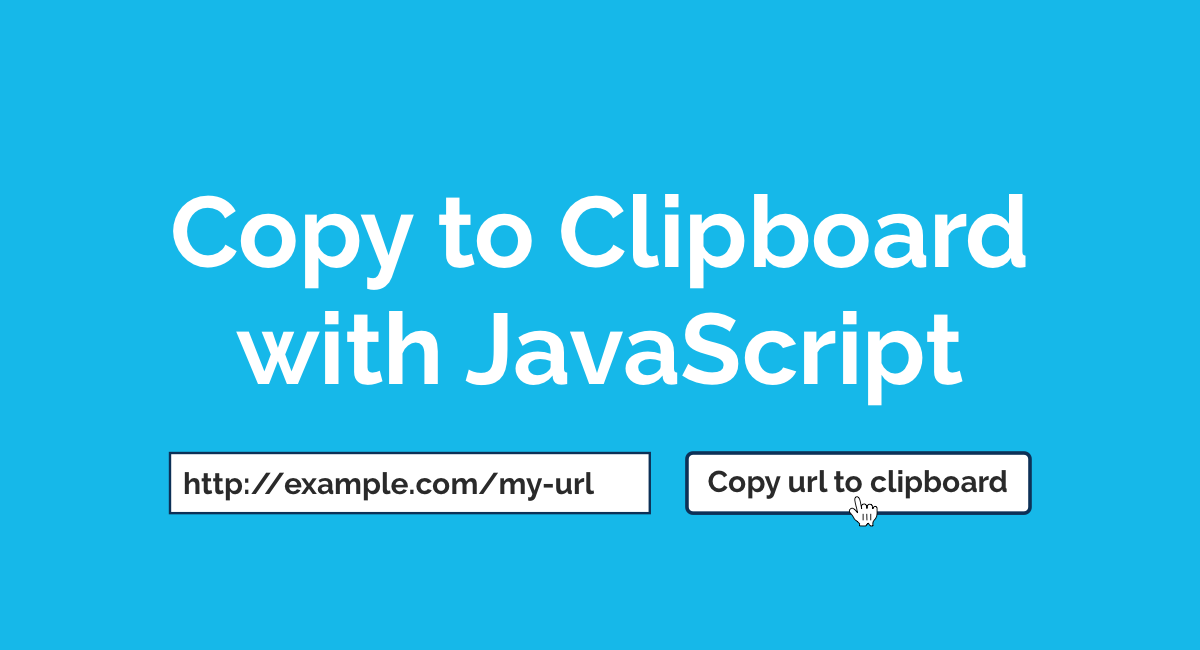The image features a light blue square-shaped background, designed to provide instructions related to copying text to the clipboard using JavaScript. Prominently displayed in the center of the image is the instructional text "Copy to Clipboard with Javascript," written in white with specific capitalization - "Copy," "Clipboard," and "Javascript" all starting with uppercase letters, and "Javascript" written as a single word.

Beneath this central text, there are two distinct white boxes, each with a black outline. The box on the left contains a sample website address presented in black text: "http://example.com http://my-url." This address is clearly displayed inside the white box.

Adjacent to this, on the right side, there is another white box, also outlined in black. This box features black text which reads "Copy URL to Clipboard" twice, indicating an actionable element for users to copy the provided URL to their clipboard.

Overall, the image is simple yet informative, combining instructional text with example elements to visually aid in understanding the process described.